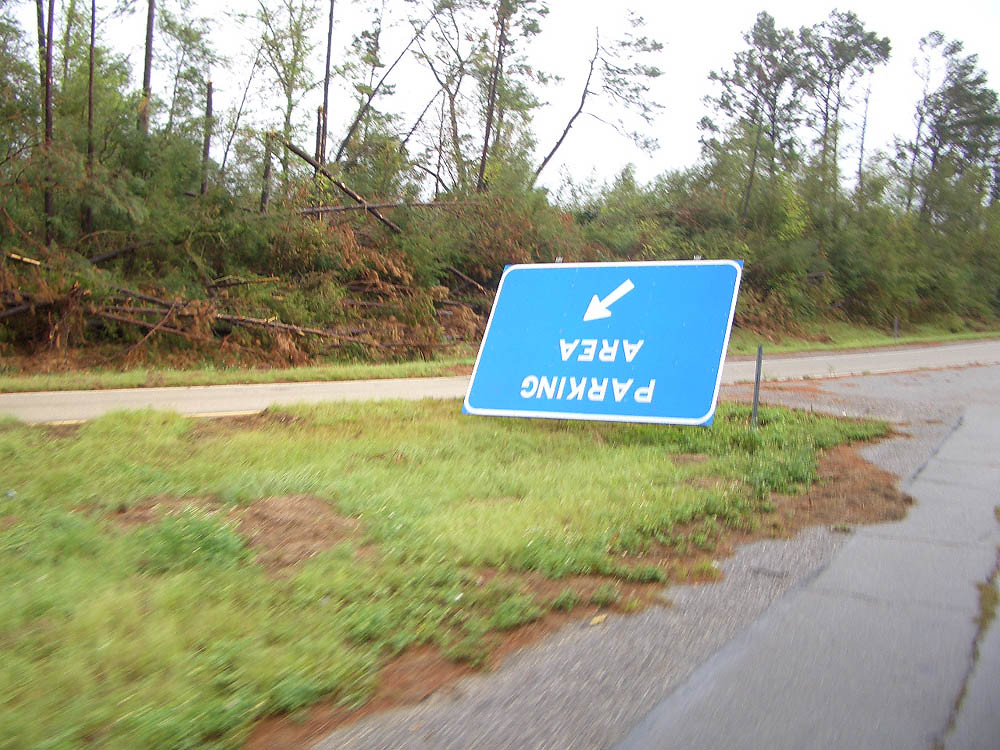In this image, an overturned sign reads "Parking Area" and points to the left. The sign, originally mounted on poles now lying broken, is situated in a grass divider between two roadways. The blue sign with white text starkly contrasts its current disarray. The background reveals several downed trees and scattered branches, indicative of recent storm damage. Mixed among the fallen trees are those still standing, sporting a mix of green and dead leaves. The road itself is littered with mud, leaves, and other debris, while the grass in the divider is torn up in patches, further supporting the likelihood of a strong storm having swept through the area.